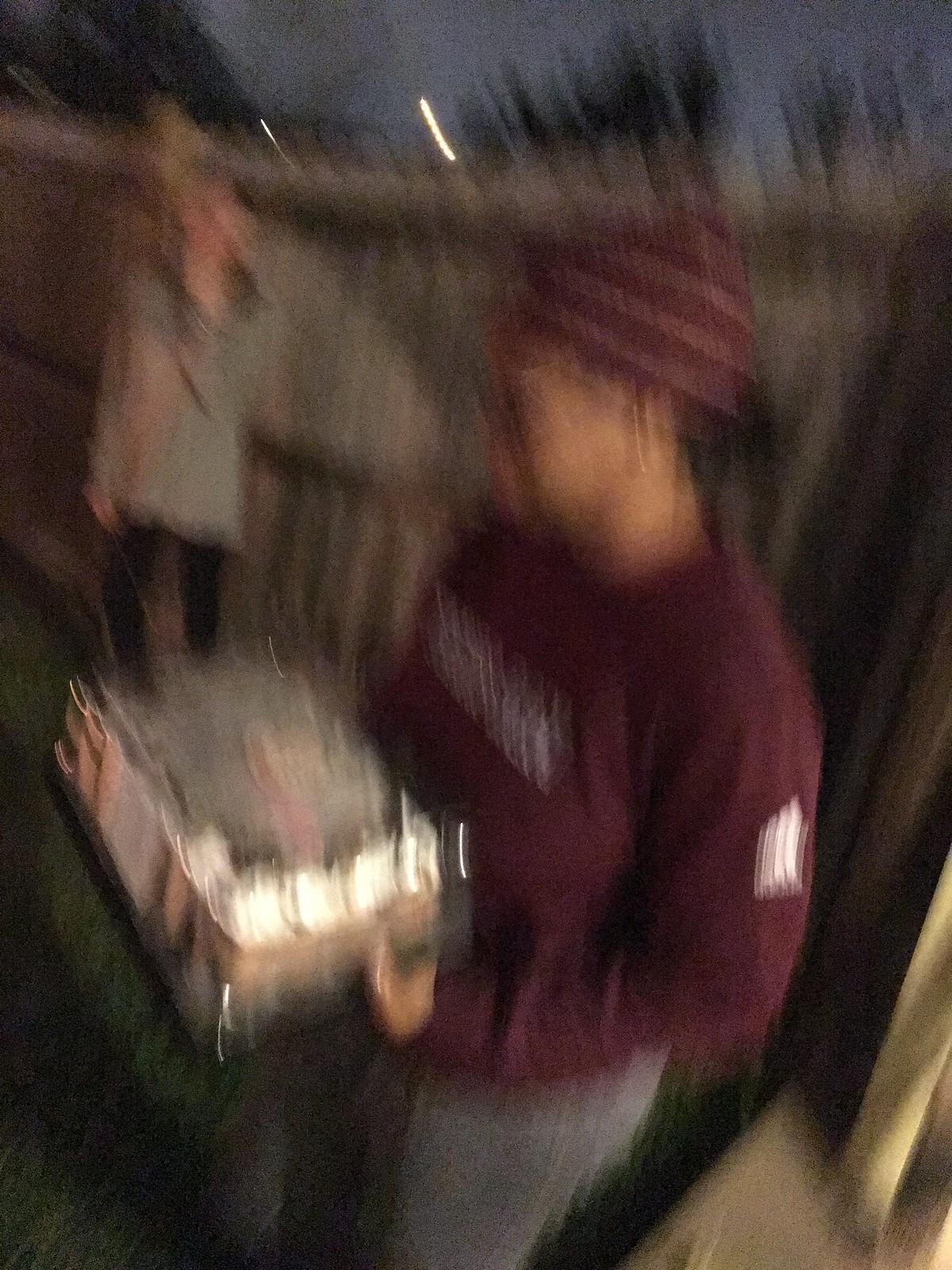In this dynamic outdoor photograph, a person is the focal point as they hold a cake, presumably celebrating a special occasion, likely a birthday party. They are dressed warmly in a burgundy and white striped winter hat and a matching burgundy sweatshirt adorned with white triangular patterns on the sleeves. Their attire is complemented by a pair of gray sweatpants. The person has a medium tan complexion, and although the white lettering on their sweatshirt's front remains indistinguishable due to the image's blur, their attire pops against the green grass underfoot. Standing behind them is another individual clad in a gray jacket and black pants, adding context to the outdoor setting surrounded by a tall, gray wooden fence. The cake in the foreground appears to be a chocolate one with a generous layer of white frosting, hinting at the festive atmosphere despite the overall motion blur that slightly obscures finer details.